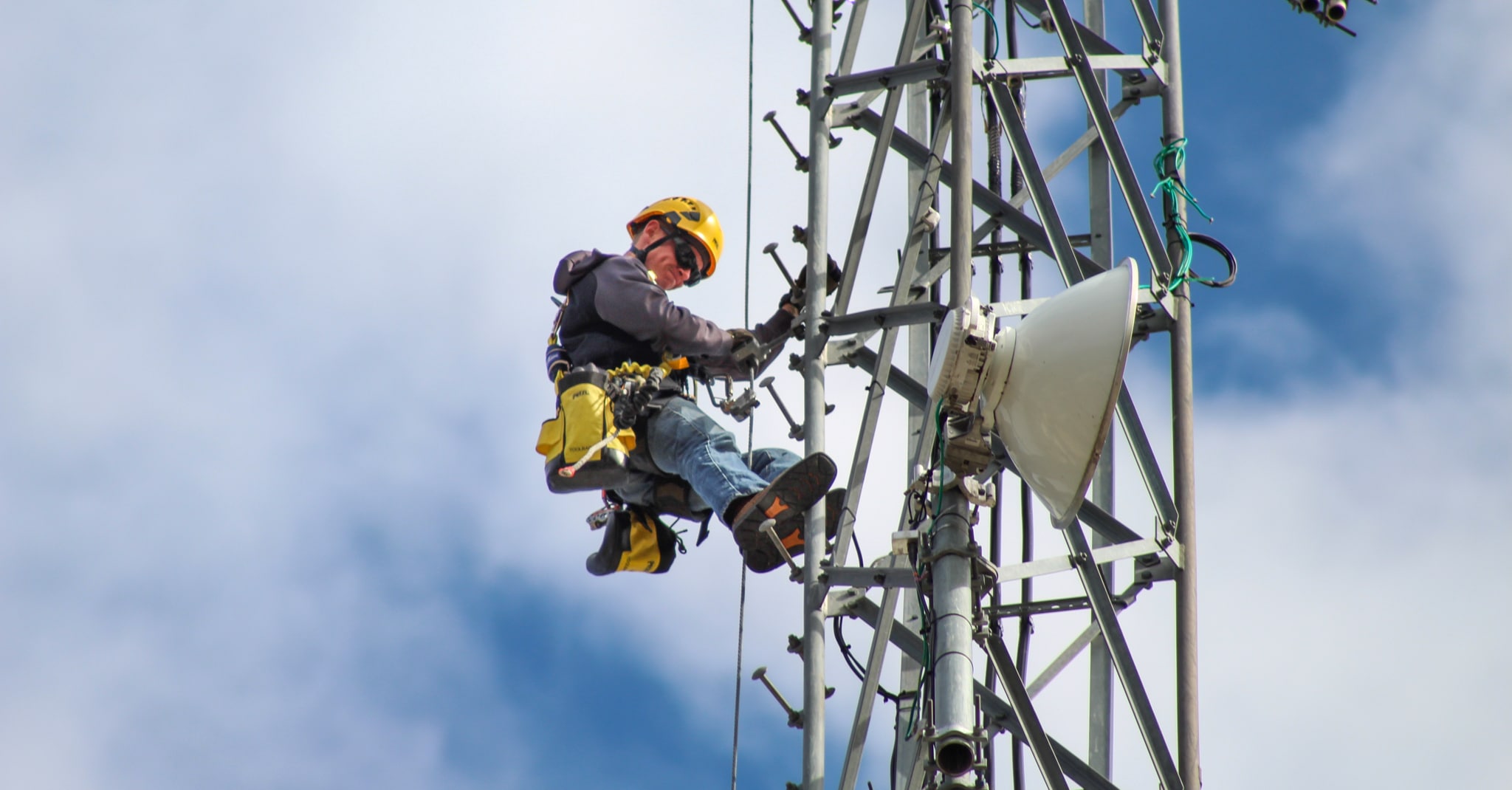In the image, we see a man positioned on a metallic scaffolding structure or possibly a cell phone tower, situated more to the right side of the frame. The structure itself is made of grayish-white, galvanized metal with a crosshatched design and extends from the top to the bottom of the image. The man, located to the left of the structure, is wearing a yellow hard hat and black glasses. His attire consists of a gray long-sleeved shirt, a tool belt with yellow details, dark-colored clothing on the top, and blue jeans at the bottom. He has various tools around his waist and his feet are firmly gripping the rungs of the tower. The soles of his shoes are distinctive, being black and orange with gray bottoms. The background reveals a vast, open sky filled with several white clouds against a blue backdrop, emphasizing the elevated perspective from which the image is taken, looking up at the man on the tower.